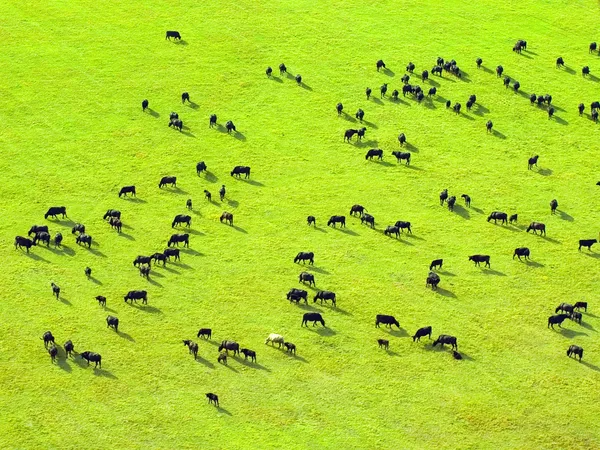This overhead rectangular photograph captures a vibrant, light green, grassy pasture abundantly dotted with cattle. Most of the cattle are black, though there are a few lighter-colored ones, possibly white cows or sheep. The cattle, including both adults and calves, are dispersed in distinct groups across the image. On the right side, clusters of cattle are visible at the top, middle, and bottom, while on the left, a large group occupies the middle with a few scattered towards the top. The lush, green grass forms a consistent background, punctuated occasionally by patches of lighter green. There is no text in the image, and all visible objects are either cattle or potentially cattle-herding dogs. Overall, the scene appears to be part of a farm or a similar outdoor setting.